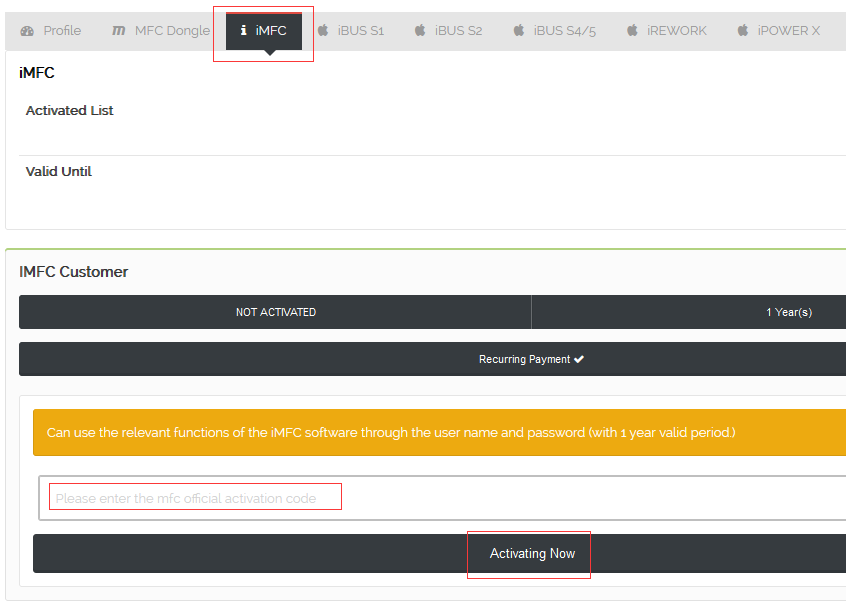This image appears to be a screenshot taken from someone's computer. At the very top, there is a gray border that features a profile icon in the upper left corner. Across to the right, there are several headings, the second of which is highlighted with a red box and darkened text, indicating it is selected. This heading reads "IMFC."

Below this, two white rectangles run the length of the screen. The upper left corner of the first rectangle is labeled "IMFC," followed by the text "activated list" beneath it. A gray line separates this section from the next, which displays the text "valid until."

In the upper left corner of the following section, a green label reads "IMFC customer." Below this label, there is a long black border stating "not activated," followed by the text "one year" to its right. Beneath that, another black border carries the label "reoccurring payment," accompanied by a white check mark.

A small white gap leads to an orange rectangle, which contains the following text: "can use the relevant functions of the IMC software through the username and password" and in parentheses it adds, "with one year valid period."

Below that, a gray box contains a red rectangle with the text "please enter the MFC official activation code." At the bottom of the screen, there is a black border that states "activating now," highlighted by a red box.